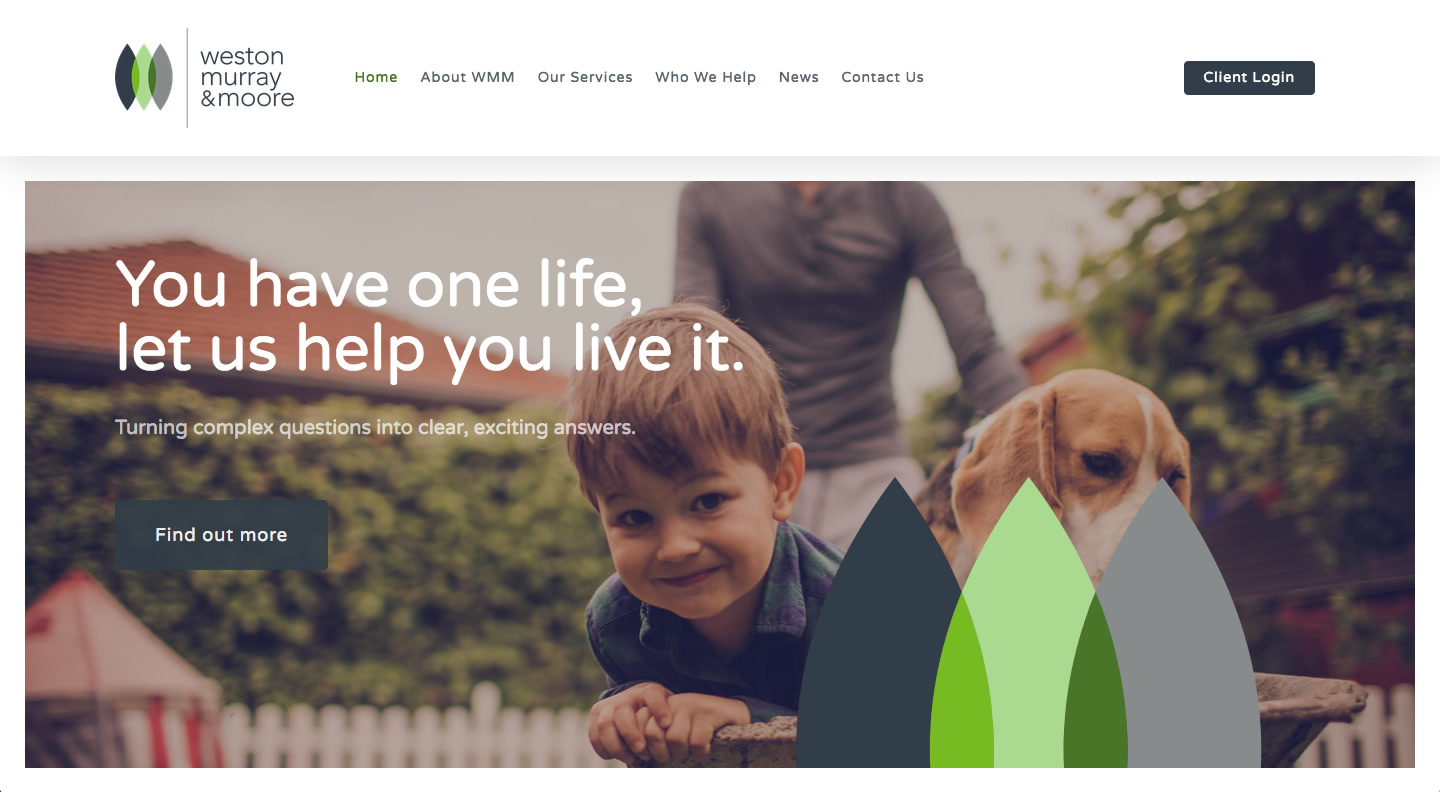The website features a clean, white background in its top portion, with the logo prominently displayed in the upper left-hand corner. The logo consists of three overlapping shapes resembling surfboards: one black, one green, and one gray. Adjacent to the logo, a dividing line separates it from the company name, "Western Murray & Moore," which is written in lowercase letters. 

The navigation menu spans from left to right and includes six options: Home, About WMM, Our Services, Who We Help, News, and Connect Us. In the far right-hand corner, there is a black button with white text that reads "Client Login."

Below this upper section, a very light, semi-transparent gray border runs horizontally. Beneath this border lies an image with white text overlay in the upper left corner that reads: "You have one life. Let us help you live it, turning complex questions into clear, exciting answers." A greenish-black box with white text beneath the overlay says, "Find Out More."

The featured image depicts a sunlit yard scene. In the background, there is a tiled roof of a neighboring house and a tall, green hedge providing privacy, along with a white picket fence. A nearby triangular awning can also be seen. In the foreground, a young Caucasian boy with a mop of brunette hair is smiling while holding the edge of a wheelbarrow. Inside the wheelbarrow is a beagle with brown floppy ears, brown fur on its head, a white stripe running down its face, and a white snout. The wheelbarrow is being pushed by an individual, presumably the father, dressed in tan-colored pants or shorts and a gray long-sleeved shirt, though their face is not visible. Over the dog's face, the company's logo—featuring the black, green, and gray surfboard shapes—appears as an overlay.